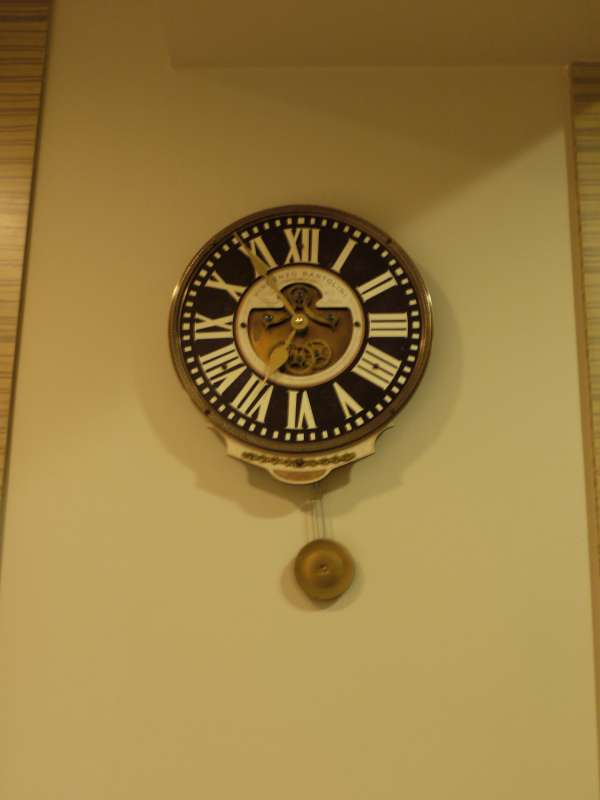This is an image of a round wall clock prominently displayed on a section of a dingy yellow wall. Flanked on both sides by wooden panels, the contrast between the worn yellow section and the rich wooden texture is striking. The clock is encircled by a brass-colored ring, adding a touch of elegance to its design. Its face is a deep black, adorned with white Roman numerals and minute markings, providing a stark contrast for easy readability. At the center of the clock, a white area features a decorative brass element. Both the hour and minute hands, also brass, accentuate the clock's vintage appeal. The minute hand is pointing just shy of the 11 at 55 minutes, while the hour hand rests at 7. Below the clock face, a pendulum swings, adding a dynamic touch to the otherwise static timepiece.